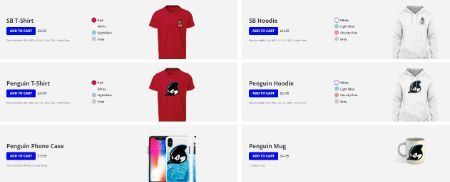This image appears to be a small and difficult-to-read screenshot likely taken from an online store. The site offers various penguin-themed merchandise, including t-shirts, hoodies, mugs, and phone cases. The graphic designs of the products are simplistic and seemingly of inconsistent quality, hinting at a mass-produced nature typical of print-on-demand websites. The background is plain white, adding to the underwhelming visual appeal. This type of store, which may be similar to platforms like Redbubble, often focuses on maximizing profit by applying generic images to a wide range of merchandise with minimal attention to design excellence or uniqueness.